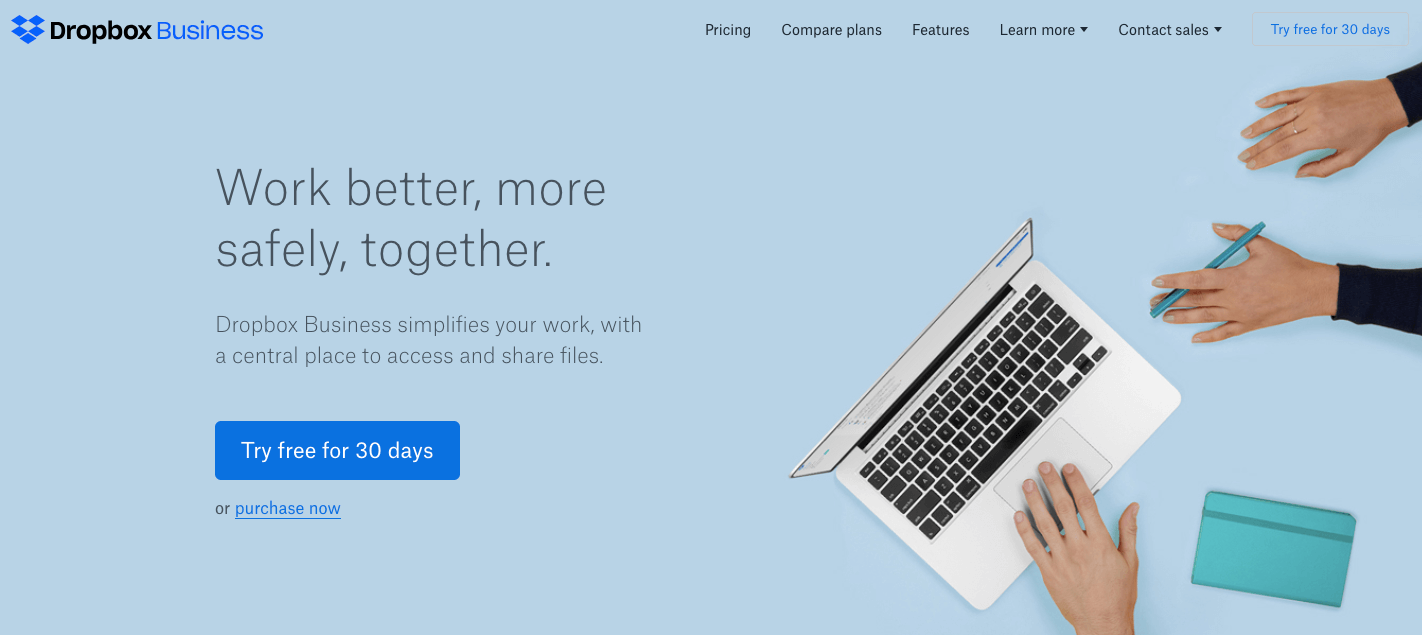A detailed screenshot of the Dropbox Business homepage is displayed. In the top left corner, there's the Dropbox logo in blue with the word "Business" also in blue. The website's main navigation bar across the top has options in black text: "Pricing," "Compare Plans," "Features," "Learn More," and "Contact Sales." 

Prominently, a blue button with the text "Try free for 30 days" stands out, along with a motivational slogan in large font: "Work better, more safely together." Below this, a subtitle reads, "Dropbox Business simplifies your work with a central place to access and share files."

Further down, there's another blue button labeled "Try free for 30 days" and a link for purchasing now in blue text. The website aims to give a modern, professional feel, which is enhanced by an image on the page. 

The image features a blue backdrop resembling a tabletop. On the table, there's a MacBook viewed from above, with a hand resting on the keypad. Next to the MacBook, there’s a blue notebook. In the upper right corner, a pair of women's hands, wearing a black long-sleeve shirt, hold a pen, suggesting productivity and collaboration in a modern business environment.